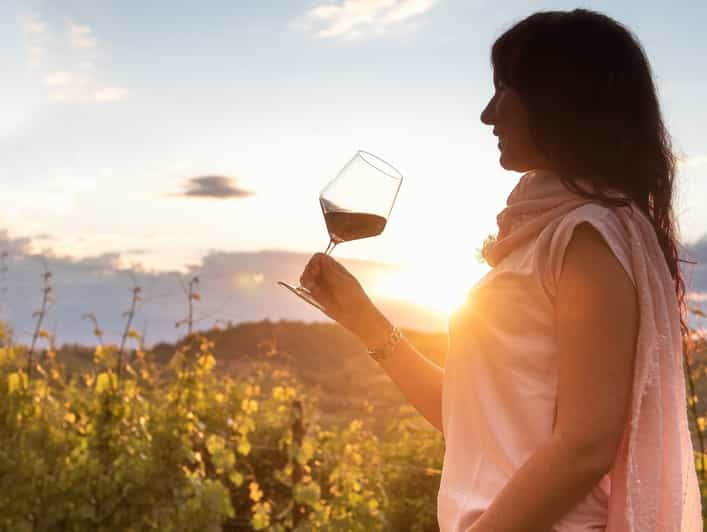In this captivating photograph, a young woman is seen enjoying a glass of wine while standing in a lush vineyard at sunset. She is positioned in profile, facing left, with her long, dark hair flowing down her back. The light from the setting sun casts a warm, orange glow on the scene, creating a serene and picturesque atmosphere. The woman is wearing a light pink scarf wrapped around her neck and a sleeveless pink shirt that beautifully complements her outfit. A gold bracelet adorns her hand as she delicately holds a large, opaque wine glass containing a rich, dark red wine, tilted slightly towards her lips.

The background reveals a vibrant vineyard, with grapevines stretching on either side of her, a mix of green and yellow leaves glistening in the sunlight. Supporting posts can be seen amongst the grapevines, adding structure to the natural setting. Behind the vineyard, a modest hill rises, partially covered by thick, gray clouds that linger just above it. As the eye travels upward, the sky transitions from the dense cloud cover to a clearer blue expanse with only a few wispy clouds. Beyond the hill, dark green mountains add depth to the landscape, enhancing the overall sense of tranquility and natural beauty in this evening shot.